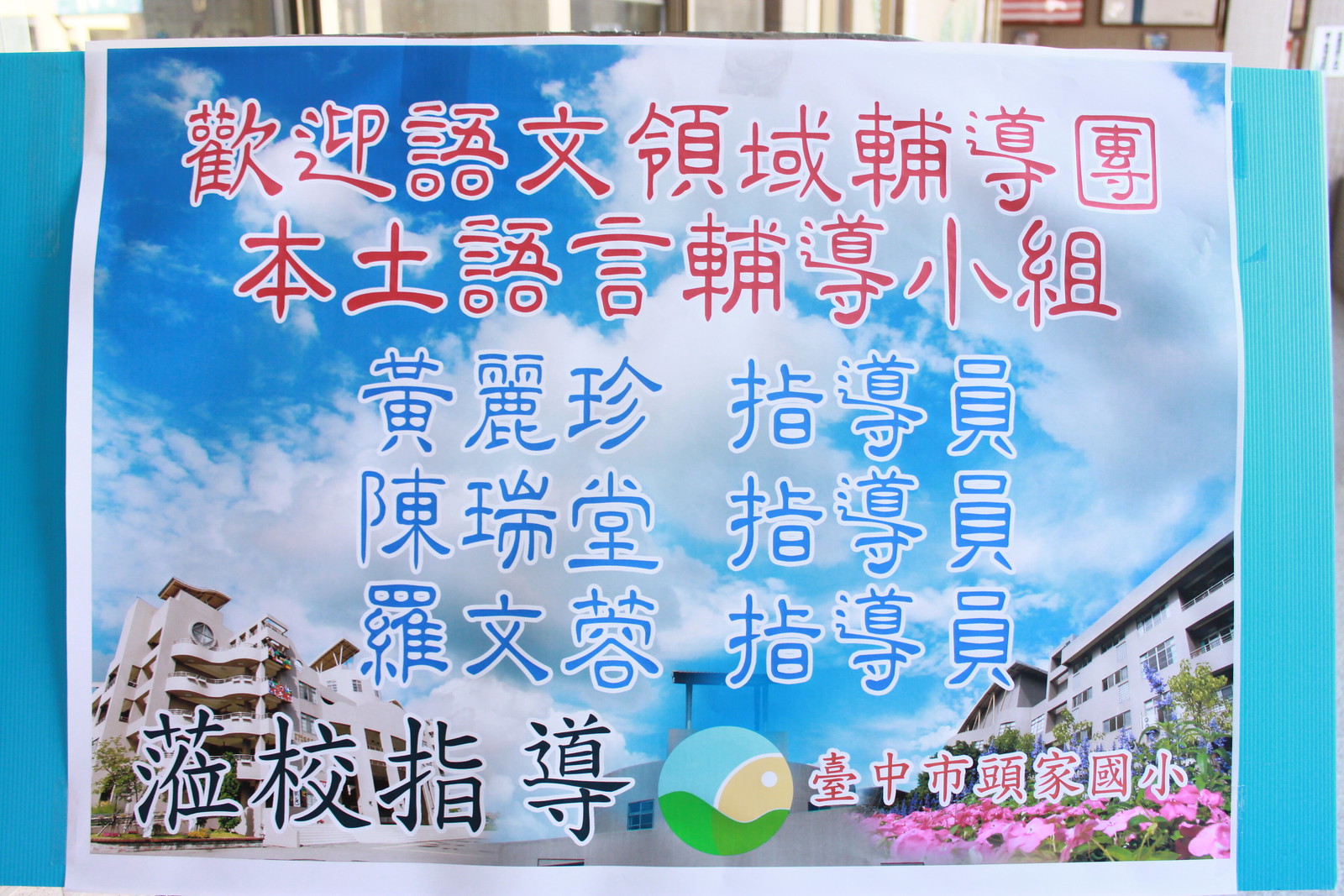The image appears to be an advertisement featuring a daytime outdoor scene, framed by a light blue border on both sides. Dominating the foreground are two white buildings: one on the left, a tall residential complex with about four to five stories and balconies; and another shorter building on the right, lacking balconies but adorned with shrubbery, flowers, and possibly indicative of a vacation resort or smaller apartment building.

The backdrop boasts a beautiful blue sky dotted with clouds, and there is a distant sight of a stadium marked by a scoreboard further down the middle background. At the center of the image, Chinese or Japanese text written in red extends horizontally from left to right, flanked by additional blue text arranged vertically. The very bottom of the image features more text in smaller characters: black on the left and red on the right, with a complex logo in the center, which includes green and blue elements resembling a sun setting over land. The entire layout suggests an ad promoting a particular location, highlighted with character lettering and various scenic elements.